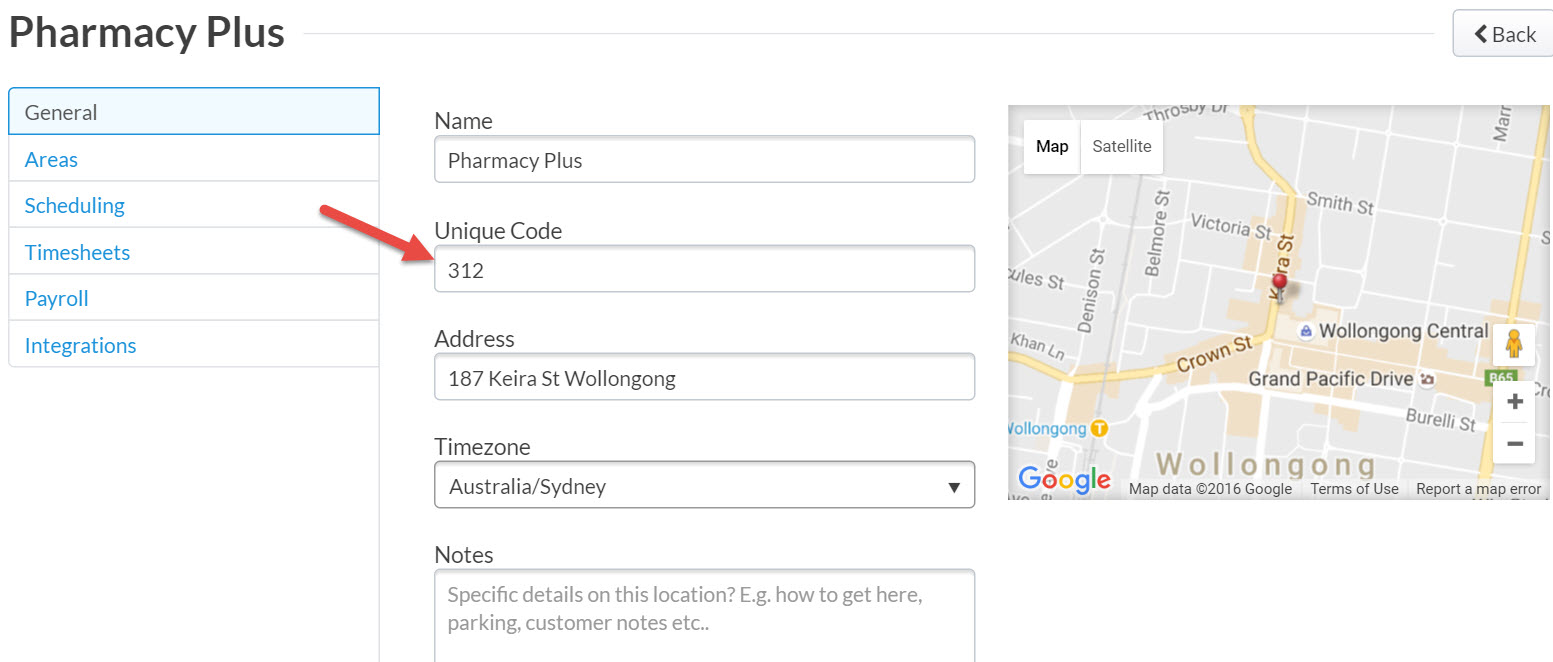The web page for the company "Pharmacy Plus" is displayed prominently, with the company's name in large, bold black lettering situated in the upper left-hand corner. All text on the page is either in black or gray, unless specified otherwise. Directly below the "Pharmacy Plus" title, there are menu options listed vertically in blue lettering: "General," "Scheduling," "Timesheets," "Payroll," and "Integrations." 

To the right of these options, there are search functionalities marked by a red arrow pointing to "Unique Code 312." This section includes search fields for "Name," where you can look up "Pharmacy Plus," "Unique Code 312," "Address" at "187 Kiara Street, Wollongong," and "Time Zone" set to "Australia/Sydney." Additional notes provide specific details about this location, including directions, parking information, and customer notes.

A map program, utilizing Google Maps, is displayed prominently on the page, pinpointing the exact location of the shop. In the upper right-hand corner, there is a large "Back" button designed to navigate users back to the previous page. This webpage appears to be a navigational tool for finding businesses and generating route information.